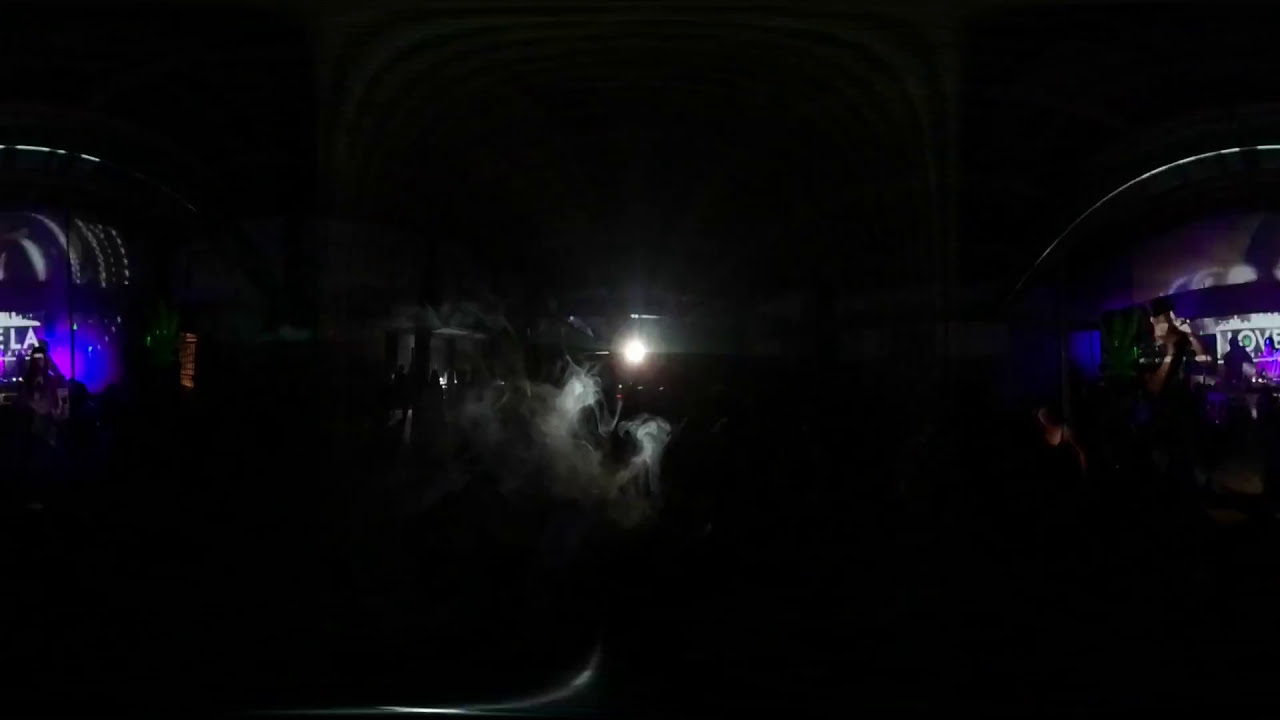The image seems to be taken in a dimly lit studio or stage setting, possibly at an event like a Coachella music festival. The center of the image is enveloped in darkness with only a small light source and some smoke rising from the ground, making it difficult to discern specific details. On the right side, shadows reveal people standing, potentially around a desk with computers or similar equipment, against a backdrop that features white shelving adorned with the word "Love" and a sculptural element above it. The left side displays a glass panel backlit with blue and pink-purple tones, hinting at a stage or set piece. Partial letters "ELA" are visible, which might correspond to "Coachella" or a similar event. The arrangement suggests a busy environment with multiple light sources and possibly people working in the background. Overall, the setting combines the elements of a sophisticated studio or a concert stage, with dim lighting, accented by colorful lighting and scattered details.